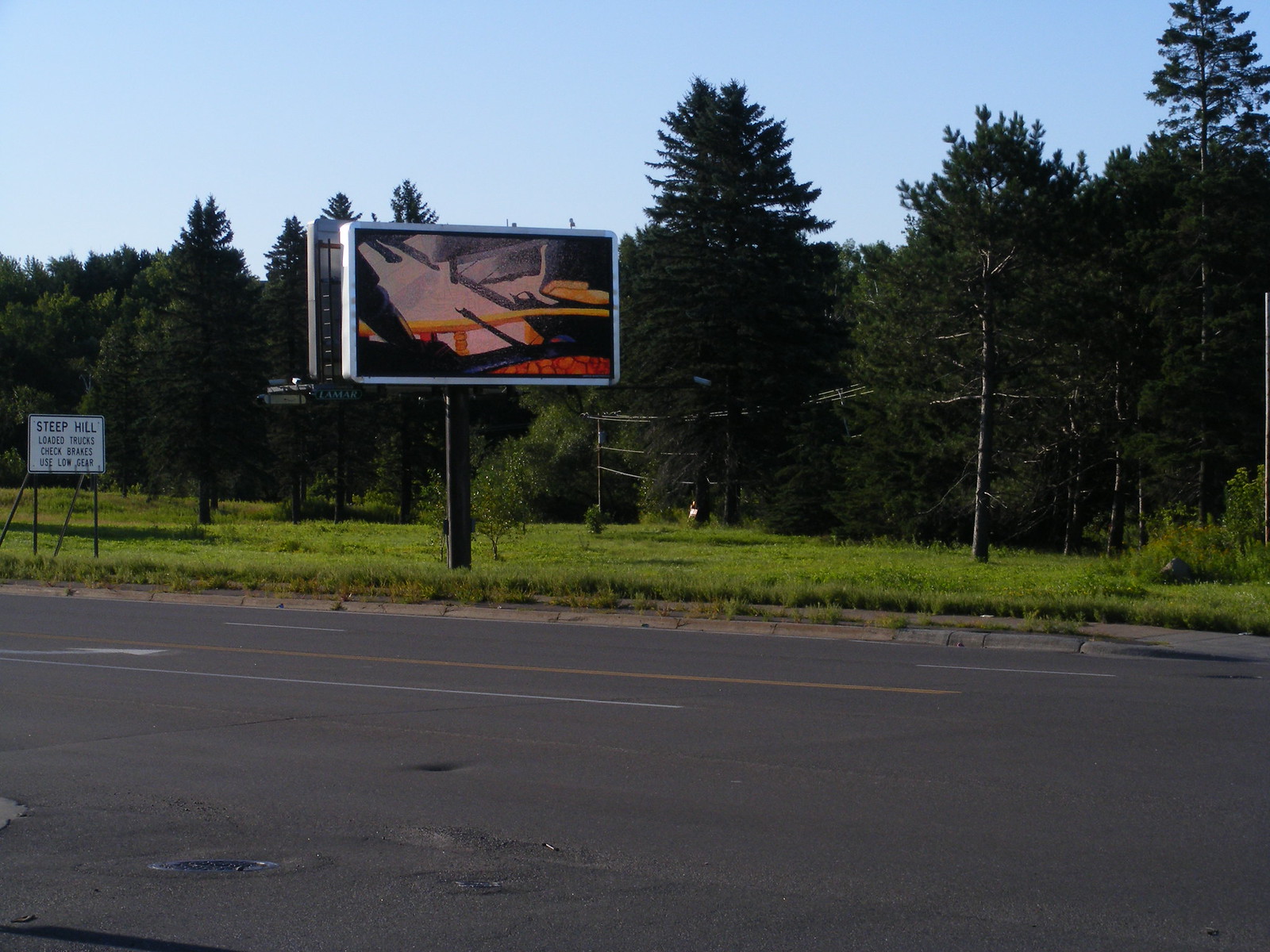This photograph captures a scenic roadway bordered by a verdant stretch of grass. Positioned prominently on the grassy verge is a large billboard featuring an abstract artwork. The piece displays a harmonious blend of colors, predominantly orange and yellow. The orange section reveals a marbled texture, while a yellow area appears to form a railing-like stripe across the middle of the billboard. Additional hues of gray and black are interspersed throughout the composition, contributing to the artwork's abstract and non-representational nature. The entire scene evokes a sense of modern artistry juxtaposed against the simplicity of the natural roadside.